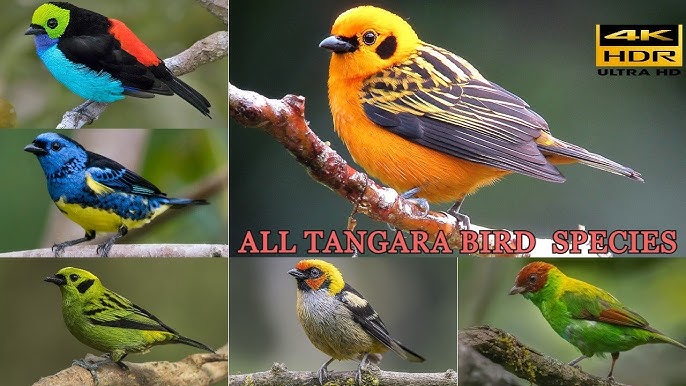The image is a montage showcasing six photographs of Tangara bird species, highlighting their vibrant diversity. 

In the larger, top-right frame, a stunning bird with a predominantly bright orange body and dark gray wings and tail is featured. Its head is mostly orange with a touch of black on the side and a small black beak.

The top-left photo depicts a highly colorful bird with a blue chest, a green head, black wings, and tail, with a bright red patch on its back, perched on a gray branch.

Directly below, the middle left photo shows a bird with a blue body, yellow chest, and black accents on its wings, also sitting on a gray branch. 

The bottom left picture captures a mostly lime-green bird with black accents and speckles on its wings, perched on a brown branch.

In the center bottom, a bird with a gray body, a distinctly yellow and orange face, and black wings is displayed, standing on a gray branch.

Lastly, the bird in the bottom right corner has a green body, a red head, brown wings, and an orangish-red splash on its wings with a splash of yellow on its back, perched on a brown branch.

All the perched birds have gray feet and small black beaks. Text on the image reads “All Tangara Bird Species,” with a logo in the upper right corner stating “4K HDR Ultra HD.”